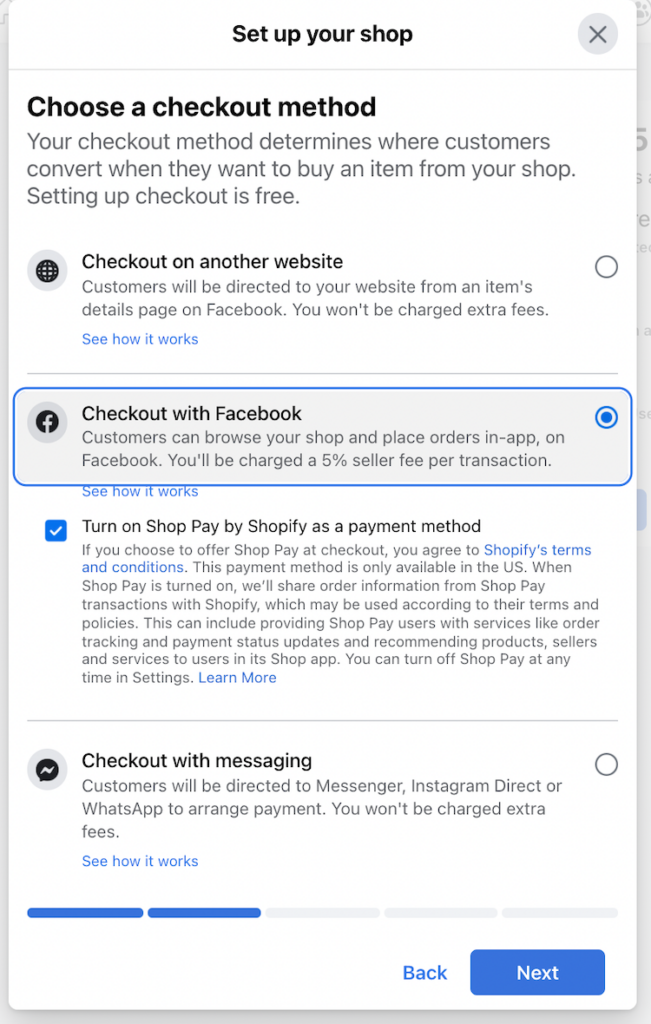The screenshot depicts a setup interface for configuring an online shop on a mobile device. At the top, in prominent black font, it displays the prompt, "Set up your shop," alongside an option to "X" out or close the setup. Below this, the heading "Choose a checkout method" is highlighted in bold, signaling an important step in the setup process. 

A brief explanation follows, stating: "Your checkout method determines where customers convert when they want to buy an item from your shop. You can set it up and say, this is free." This is succeeded by a series of options for checkout methods:

1. **Check out on another website:** Customers will be directed to your website from an item's details on Facebook, with no additional fees charged for this redirection. An option is provided to "see how it works."

2. **Check out with Facebook (highlighted):** Customers can browse your shop and place orders directly within the Facebook app. A $5 seller fee per transaction applies. There is also an option to see more details about this feature.

The currently selected option includes a prompt to "Turn on Shop Pay by Shopify" as a payment method. The selection of this option implies agreement to the terms associated with Shop Pay. Additional details and terms can be reviewed by the user.

3. **Check out with messaging:** Customers will be directed to Messenger, Instagram Direct, or WhatsApp to arrange payment. This is another versatile method available for customer transactions.

The user is currently viewing the details for using Shop Pay by Shopify and appears to be considering enabling this feature despite potential associated fees. The concise explanatory text and clearly presented options are designed to guide the user through choosing the most suitable checkout method for their online shop.